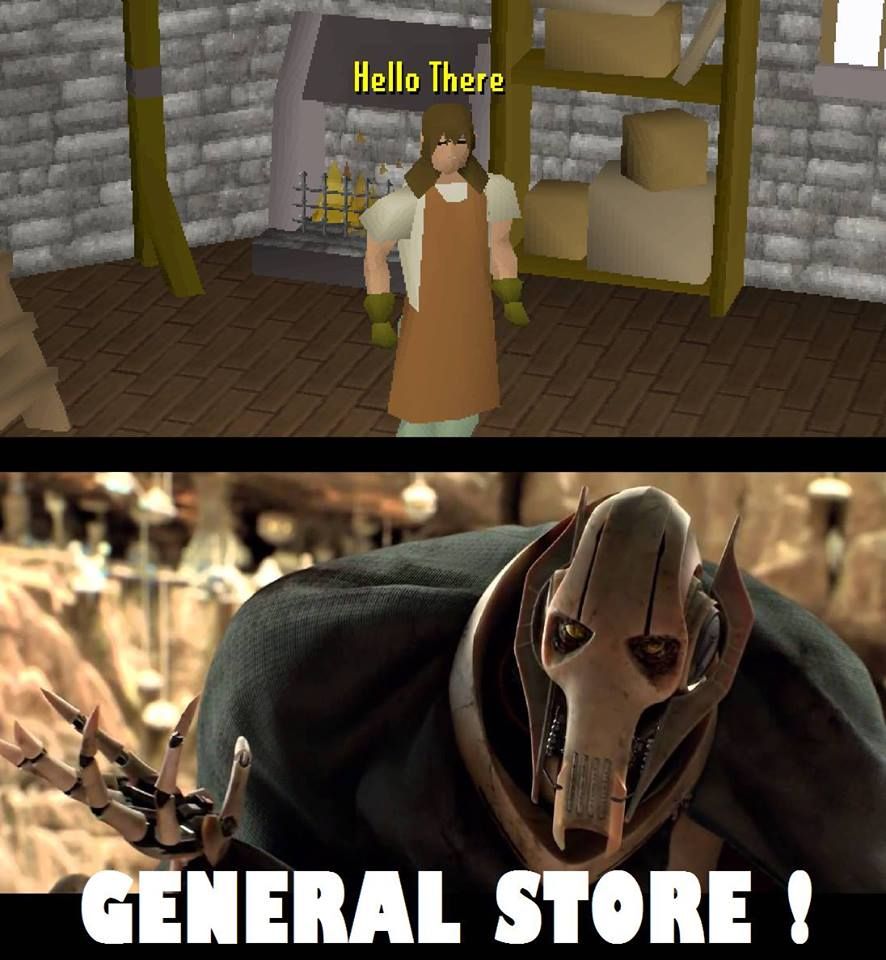The composite image consists of two computer-generated scenes positioned vertically. The top image features a female character with shoulder-length brown hair, a brown jumper dress with white sleeves, and green gloves. She stands in the middle of a room with gray brick walls and a brown brick floor. Behind her, there is a brick fireplace and a shelf with brown boxes. Above her head, in yellow font, are the words "Hello there." The bottom image depicts an alien creature with a skeletal, elongated face, big black eyes, and long, claw-like fingers. The creature is clad in black clothing, set against a backdrop that resembles rocky terrain and buildings reminiscent of Star Wars. In large, bold white letters at the bottom, it reads "General Store!"